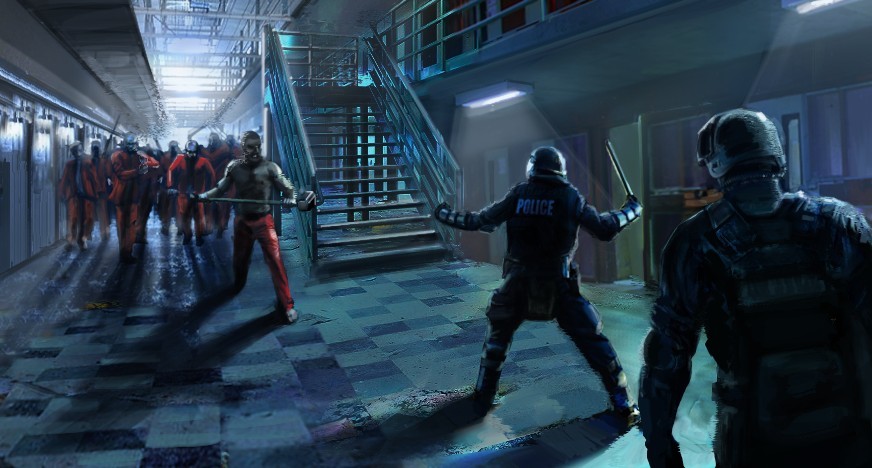This image is a highly detailed 3D digital rendering, possibly AI-generated, depicting a dramatic and tense scene within a prison. Central to the image are two police officers in full riot gear, wearing bulletproof vests and helmets, with one officer gripping a baton. The word "POLICE" is clearly visible emblazoned across the back of one officer's vest. The officers stand on the right-hand side, facing an imminent threat from a group of prisoners who are ominously approaching from the left. The prisoners are depicted in high volume on the lower level, wearing orange prison jumpsuits and wielding makeshift weapons, suggestive of a chaotic uprising.

The scene is lit dramatically with lighting streaming from a skylight above, creating stark contrasts and casting deep shadows that add to the foreboding atmosphere. Fluorescent lights contribute to the murky, backlit environment. A large steel staircase dominates the center of the image, leading up to a second level that encircles the prison, complete with a landing. The floor of the lower level features a striking black and white checkered pattern, complementing the dark, oppressive mood of the piece. The most terrifying aspect of the image is the impending confrontation, as the outnumbered officers brace themselves against the advancing, armed prisoners, one of whom is prominently featured in the foreground, shirtless and holding weightlifting equipment while sneering menacingly.